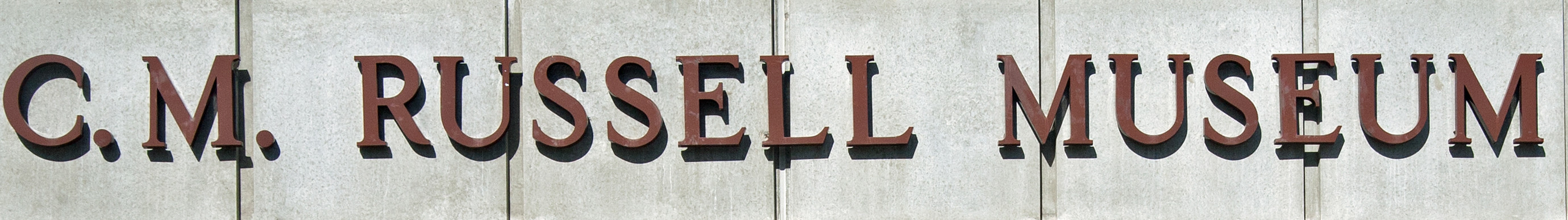This photograph captures the sign of the C.M. Russell Museum, prominently displayed on the exterior of the museum building. The sign features a rustic, brownish-red font that gives it a vintage and weathered appearance. It is affixed to a wall with notable vertical creases that align precisely with certain letters in the sign. These creases occur at various points: at the "M" in "C.M.," between the "U" and "S" in "Russell," as well as through the "L" in "Russell," the "M" in "Museum," and finally the "E" in "Museum." The detailed placement against the lined wall adds a unique texture and visual interest to the sign, blending harmoniously with the building's aesthetic.